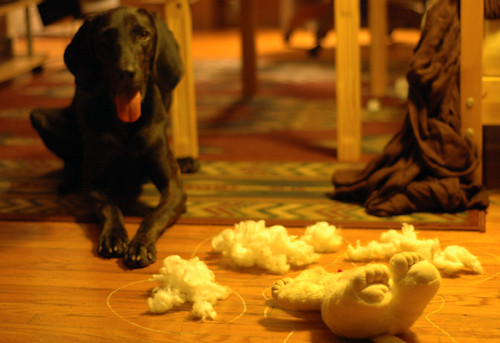This photograph captures a black dog, likely a lab or Weimaraner, laying on its belly on a large area rug. The setting appears to be inside a house, underneath a table or chairs, as the wooden legs are visible but the rest of the furniture is not. The dog is facing the viewer with its front paws outstretched, one ear raised and the other flat, looking at the camera with its tongue hanging out. In front of the dog, to the left, lies a cream-colored stuffed animal, possibly a bear, with its stuffing scattered around it in several large piles. Interestingly, the stuffed animal and the stuffing are outlined in chalk lines, evocative of a crime scene. The scene is set on a light-colored wooden floor with additional details like a chair leg on the right side of the photo and a blanket or cloth draped over it.